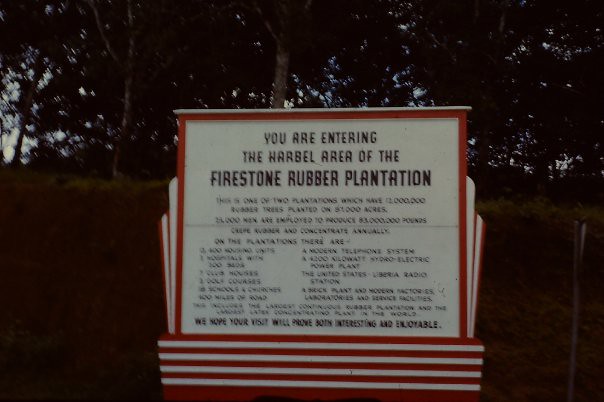The image showcases an intricate and elegant sign marking the entrance to the herbal area of the Firestone Rubber Plantation. The sign stands out with its predominantly white background and bold black lettering, clearly stating the location. The border of the sign is adorned with ornate red trim, akin to the embellishments of a movie marquee, which extends to the sides in bubble-like formations, suggesting a sense of expansion. Below the main text, the bottom portion of the sign features alternating rows of red and white stripes—five rows of each—drawing further attention to it. Though the details in the middle of the sign are not entirely legible, the concluding message at the bottom aims to ensure that visitors have an enjoyable experience. In the background, one might infer the presence of rubber trees, characteristic of the plantation.